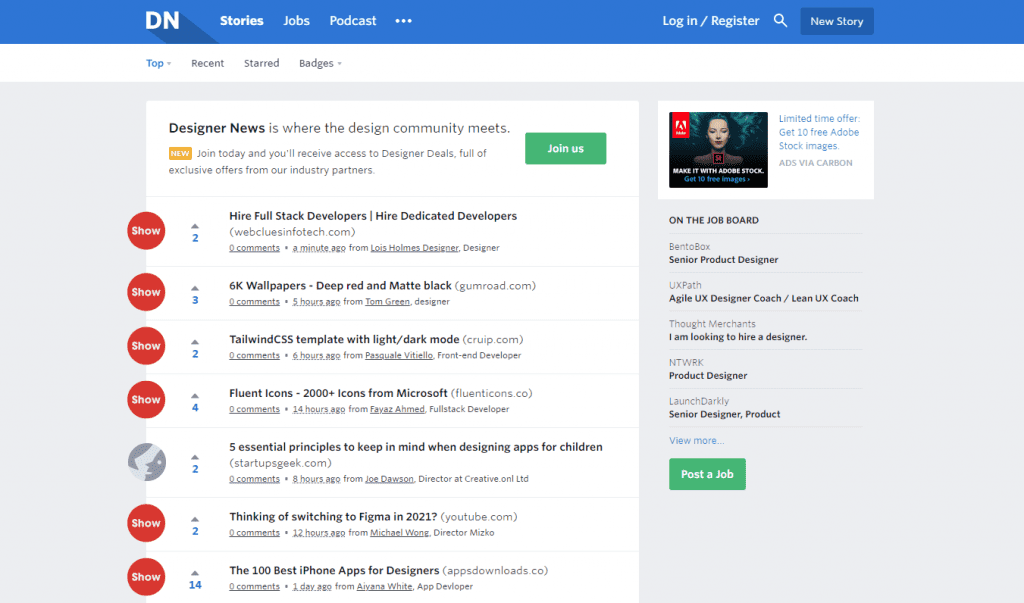On the upper left corner of the webpage, the initials "DN" are prominently displayed, indicating the site’s identity. The top navigation bar features clickable options labeled Stories, Jobs, and Podcast on the left, while Login, Register, a Search icon, and a News Story button are situated on the right. Below this section on the left side, there are four functional buttons labeled Top, Recent, Starred, and Badges.

Towards the middle left side of the page, a welcoming message states, "Design News is where the design community meets. Join Today and you'll receive access to designer deals full of exclusive offers from our industry partners." Adjacent to this message, a vibrant green button labeled "Join Us" invites users to become members.

Further down is an organized list showcasing various resources and articles:
- "Hire Full Stack Developers"
- "6K Wallpapers"
- "Tailwind C55 Template with Light & Dark Mode"
- "Fluent Icons: 2000+ Icons from Microsoft"
- "Five Essential Principles to Keep in Mind When Designing Apps for Children"
- "Thinking of Switching to Figma in 2021?"
- "The 100 Best iPhone Apps for Designers"

On the right side of the webpage, an advertisement for Adobe is displayed, providing additional visual interest and information.